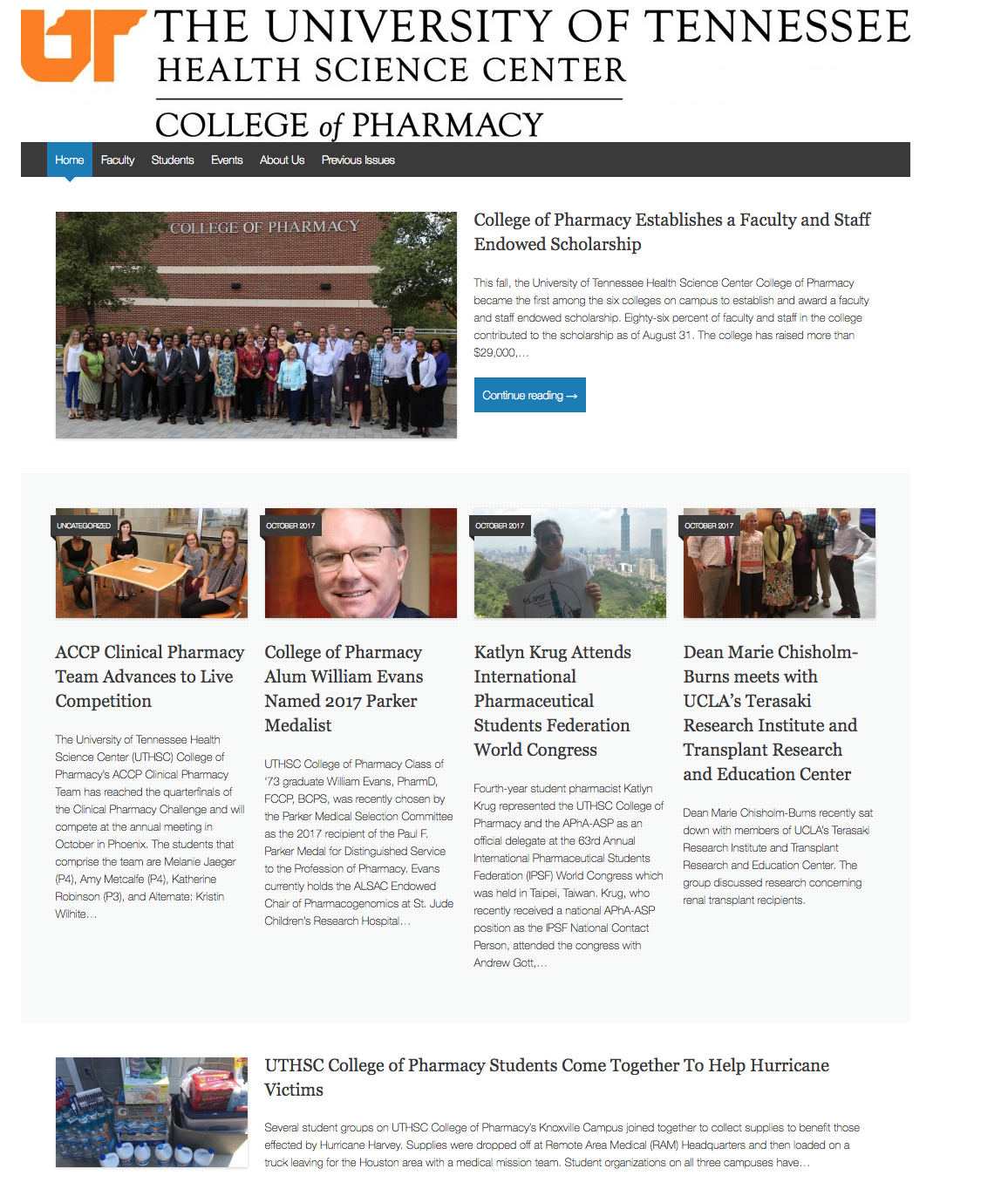This detailed screenshot captures the University of Tennessee Health Science Center's College of Pharmacy webpage. At the top, the prominent UT logo is displayed in all capital letters. Below the logo is a black navigation bar for easy site navigation.

The main section features an image alongside a headline that reads, "College of Pharmacy Establishes Faculty and Endowed Scholarship." Accompanying this headline is a descriptive paragraph and a blue button with white text inviting users to click for more information.

Further down, the page highlights four articles celebrating various accolades and achievements within the College of Pharmacy:
1. "Pharmacy Team Advances to Live Competition."
2. "College of Pharmacy's William Evans Named Parker Medalist."
3. "Pharmaceutical Students Federation."
4. "Awards Transplant."

Each of these articles has clickable links that direct readers to the full content.

At the bottom, there is a touching section about College of Pharmacy students banding together to assist hurricane victims. This includes an image showcasing the collected donations, paired with a paragraph detailing their efforts.

Overall, this screenshot provides a comprehensive view of the College of Pharmacy's initiatives, accomplishments, and community involvement.